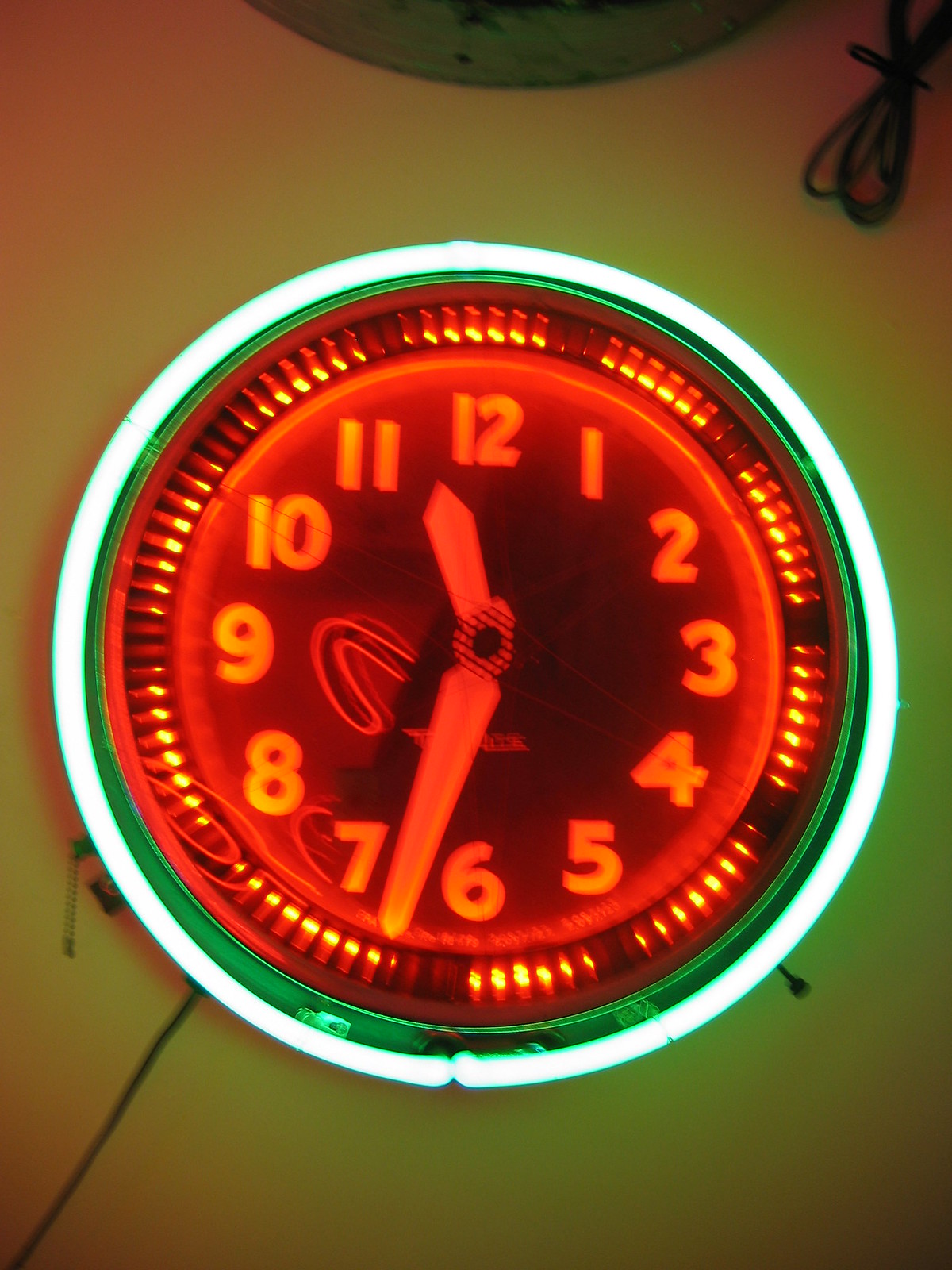The image features a brightly illuminated round clock mounted on a wall that appears yellow, likely due to light reflection in a dark room. The clock has a neon-like appearance with a wide green fluorescent rim around the outer edge and an inner bright orange or red section, creating a vivid contrast. The clock face displays large numbers from 1 to 12, with wide and large orange hands indicating the time as approximately 11:30. The clock is plugged in, with a cord stretching down from the bottom left corner. Additional details include a folded cord at the top right and a partial view of a round image at the top center. The overall design is a mix of contemporary illumination and classic analogue time display.